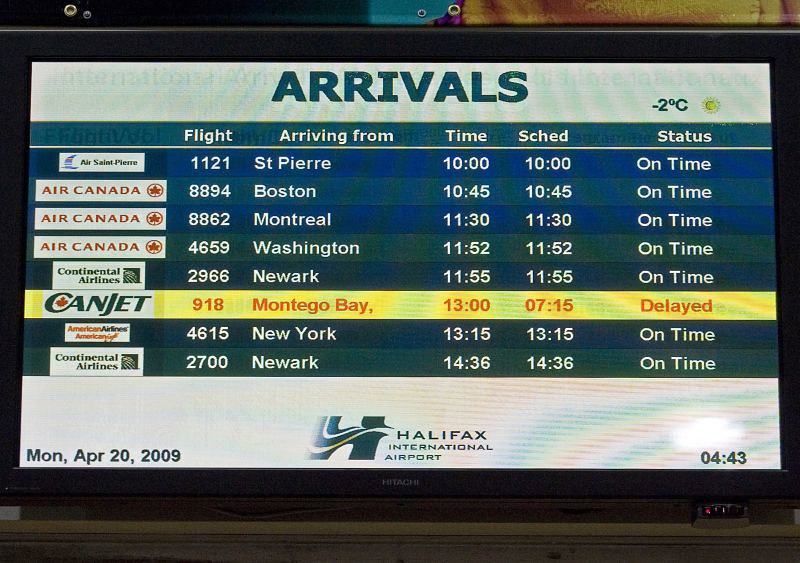The image depicts a detailed close-up of an airport arrivals screen at Halifax International Airport. The screen is organized into multiple columns providing information on various flights, including the airline name, flight numbers, originating city, scheduled arrival time, and current status. Displayed airlines include Air Canada, Air St. Pierre, Continental Airlines, CanJet, and American Airlines. The listed cities of origin for arriving flights include St. Pierre, Boston, Montreal, Washington, Newark, Montego Bay, and New York. Most flights show an "on time" status, except for a CanJet flight from Montego Bay, which is highlighted in yellow with red text indicating it is delayed. At the bottom, the screen shows the logo of Halifax International Airport along with the date and time: Monday, April 20, 2009, at 4:43 PM. The temperature is noted as negative two degrees Celsius. Additionally, a small sun icon is visible near the top of the screen.